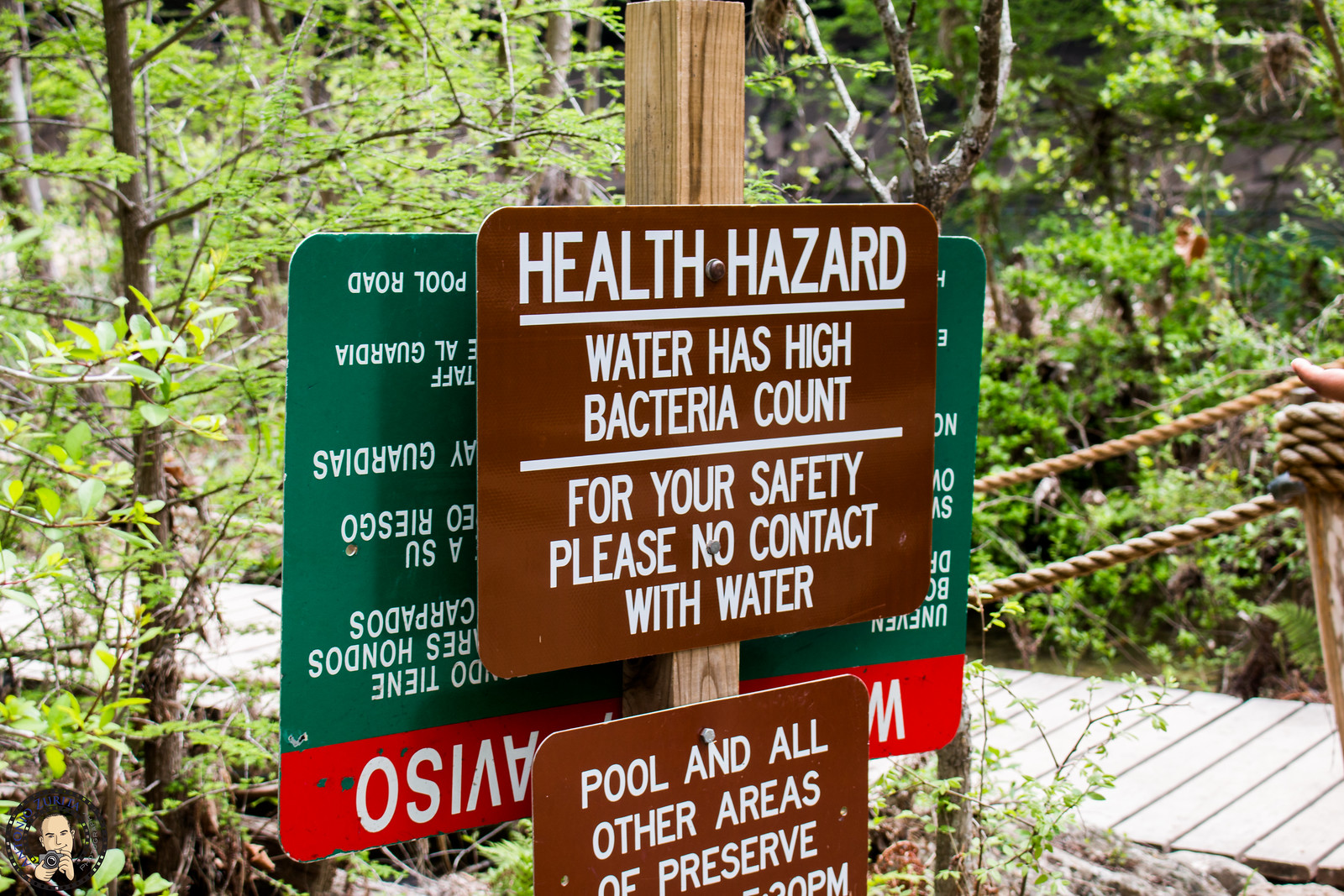The image is a detailed color photograph taken outdoors during the daytime, in a densely wooded area resembling a forest. The focal point of the image is a wooden pole, cropped at the top, situated in the center of the photograph, adorned with multiple signs. These signs include a prominent brown sign at the top that reads, "Health Hazard. Water has high bacteria count. For your safety, please no contact with water." Directly below this sign is another brown sign that states, "Pool and all other areas of preserve," followed by cut-off text indicating a specific time. There are additional signs mounted behind these, with one being upside down and displaying partially readable text such as "AVISO." The background features a wooden bridge with rope railings cutting through the greenery, which includes numerous trees and branches. Part of a hand reaching towards the bridge is also visible. Additionally, there is an illustration of a man taking a picture in the lower left corner, adding a unique, slightly incongruent element to the otherwise realistic outdoor setting. The colors in the image include various shades of green and brown, interspersed with red and white text on the signs.